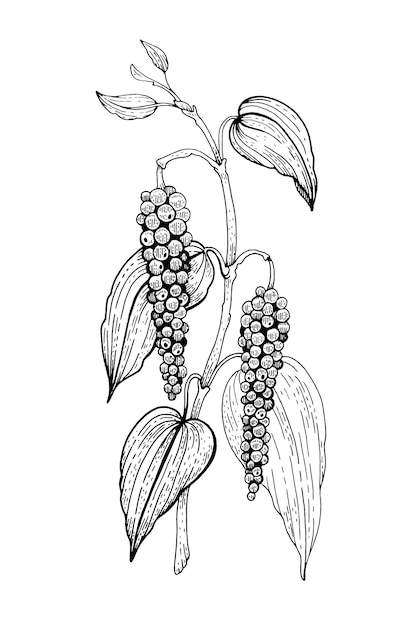This black and white, vertically oriented illustration depicts a plant with a main stem and a white, unadorned background. The plant has six distinct leaves: four large ones situated on the sides, with two on the bottom left and two on the bottom right, and two smaller leaves at the very top. The leaves are detailed with visible lines. Hanging from the stem are two clusters of round berries, likely resembling grapes, with each cluster containing approximately 20 to 30 berries. The illustration is executed with varying line thicknesses, showcasing a mix of thick and thin lines, and employs hatching techniques.